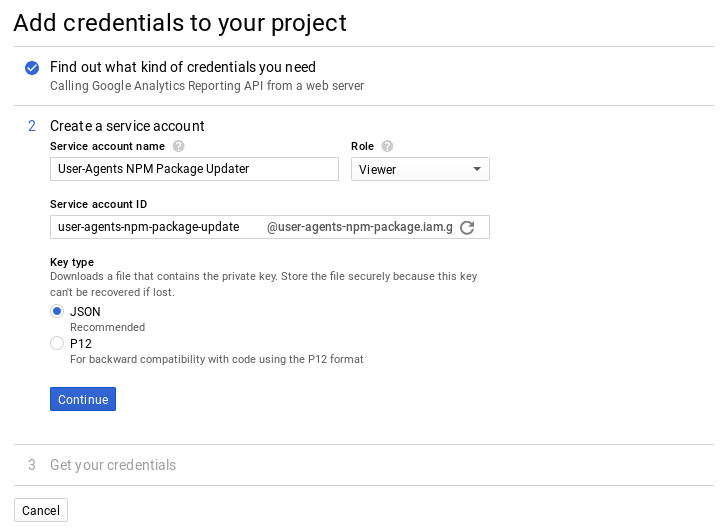The image depicts a section of a webpage dedicated to adding credentials to a project. At the top, the title "Add Credentials to Your Project" is displayed in black text. Below the title, a blue checkmark is present next to the text "Find out what kind of credentials you need," followed by details about the process for calling the Google Analytics Reporting API from a web server.

Step 2 is prominently shown, labeled with "Create a Service Account." This section includes fields such as "Service Account Name," which displays "User Agent" along with the context of an npm package update. The "Role" field is set to "Viewer," while the "Service Account ID" also reads "User Agents, npm package update." A prompt instructs to "Add User Agents, npm package, im.g" with an adjacent refresh icon.

Under "Key Type," instructions indicate the need to "Download a file that contains the private key. Store the file securely, because this key cannot be recovered if lost." Two options are provided: "JSON" (recommended and marked with a blue checkmark indicating selection), and "P12" for backward compatibility with code using the P12 format.

At the bottom, a prominent blue "Continue" button is visible, alongside a white "Cancel" button. The entire page features a clean, white background with black text for easy readability.